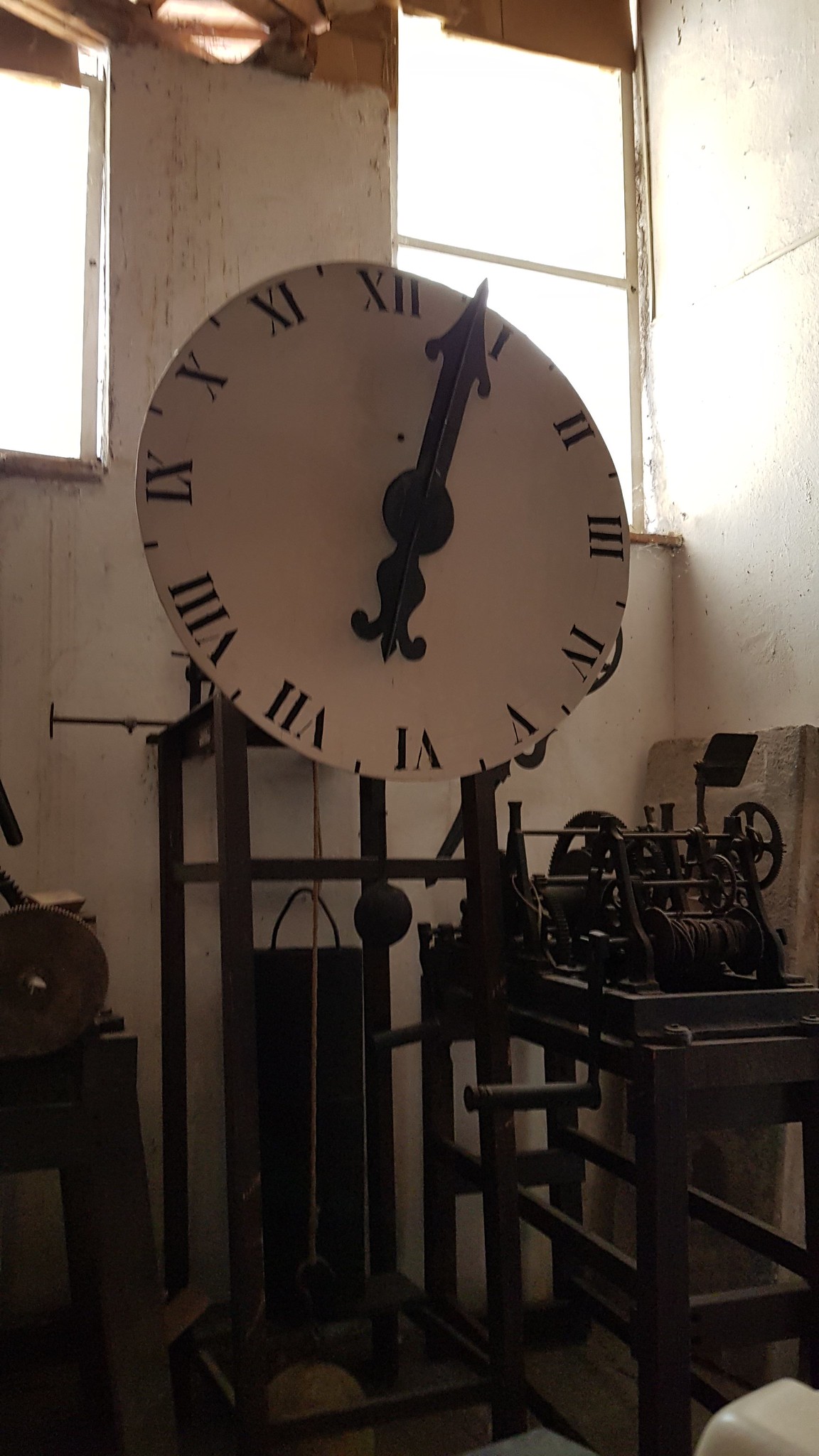This detailed photograph depicts an interior space that appears to be a workshop for large tower clocks, the type typically found in town halls or churches. The image is vertically oriented and prominently features an old clock mounted on a weathered metal stand. The clock face is large, round, and white, with black Roman numerals marking the hours. The hour hand points between 6 and 7, while the minute hand is between 12 and 1, ending in a large arrow. 

Behind the clock, a white stucco-finished wall stretches upwards, looking faded and aged. Towards the top of the image, two small, rectangular windows provide a glimpse of the outside light. These windows are positioned high on the wall, suggesting a very high ceiling and aligning approximately with where a second-floor baseline would be. 

In the foreground, there is a black metal stand under the clock, flanked by two smaller metal stands on either side. Additionally, mechanical gears and other clockwork components are silhouetted in the right center of the image, resting on another metal stand. Weights are visible hanging below the clock, enhancing the technical atmosphere of the workshop.